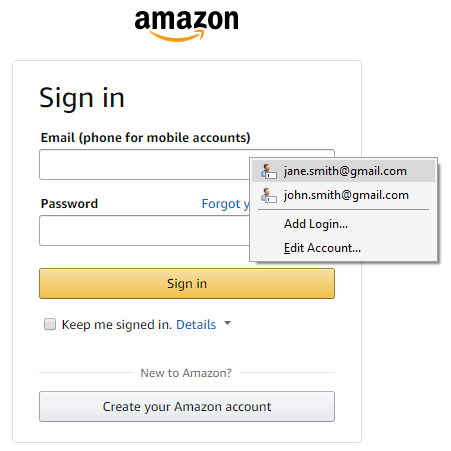The image depicts Amazon's sign-in or sign-up page. At the top of the page, the iconic Amazon logo is prominently displayed. Below the logo, there is a header saying "Sign-In." The first input field is labeled "Email or mobile phone number" and is currently empty. Some suggested email options such as "john.smith@gmail.com" appear below the input field. Next, there is a password field, which is also empty. Below the password field, a vibrant yellow "Sign-In" button is visible. There's an option to keep the user signed in, accompanied by a "Details" link for more information. Near the bottom, a prompt for new users reads, "New to Amazon? Create your Amazon account." The page is otherwise minimalistic, focusing solely on facilitating user access to their accounts.